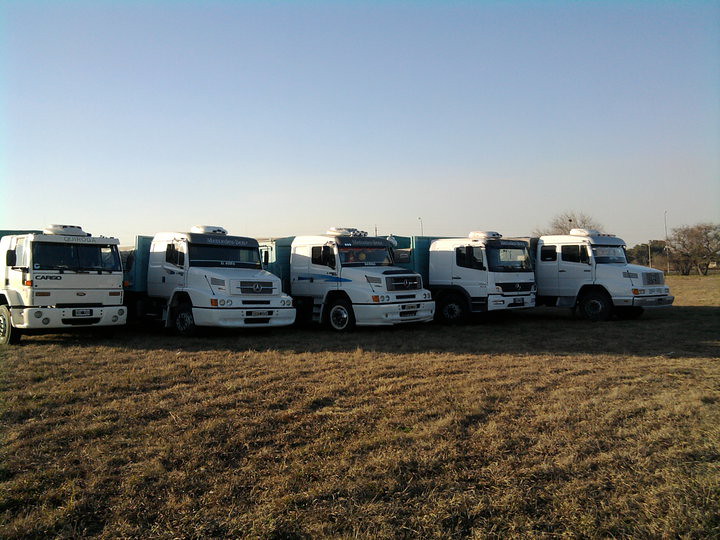The image captures five white semi-trucks parked obliquely in a row, all facing towards the lower right corner of the picture on a field of yellowish-brown grass. The trucks are a mix of cab-overs and long-nosed cabs, with refrigerator units on the roofs and green headache racks behind the cabs. They appear to be flatbeds with trailers that have a greenish or bluish tint. It's early morning or late afternoon as the sky transitions from a clear blue at the top to a hazy white lower down, indicating a sunrise or sunset. The sun is casting long shadows from the trucks towards the right side, hinting at its position in the upper left. In the background, there are some low-growing trees with few leaves and a possible pole or sign, all under the clear, cloudless sky.